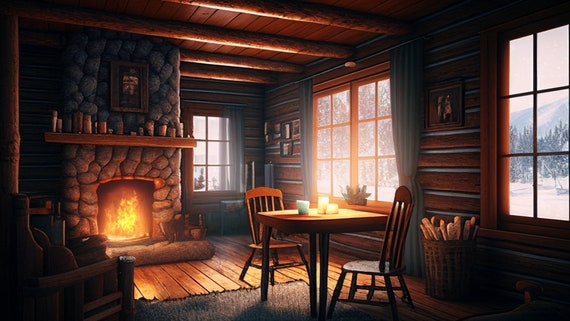The photograph displays the interior of a cozy, log cabin nestled in the mountains. The room features robust log beams supporting the ceiling and log walls that enhance the rustic charm. Centered within the space is a stone fireplace, with a roaring fire providing the primary source of illumination. Above the fireplace, a picture hangs, while the mantel is decorated with various small items, adding a personal touch to the cabin. Surrounding the room are multiple large windows, through which snowy landscapes of mountains and trees can be seen, enhancing the serene ambiance.

An easy chair sits comfortably in the lower left-hand corner, and the wood floor partially covered by a carpet adds warmth to the setting. A wooden table accompanied by two wooden chairs occupies the center of the room, with a candle and a cup placed on it. A large wicker basket filled with firewood is positioned strategically, ready to stoke the fire. Despite the darkness, the roaring fire and potentially a few lit candles on the table further emphasize the homely and tranquil atmosphere of this mountain cabin retreat.